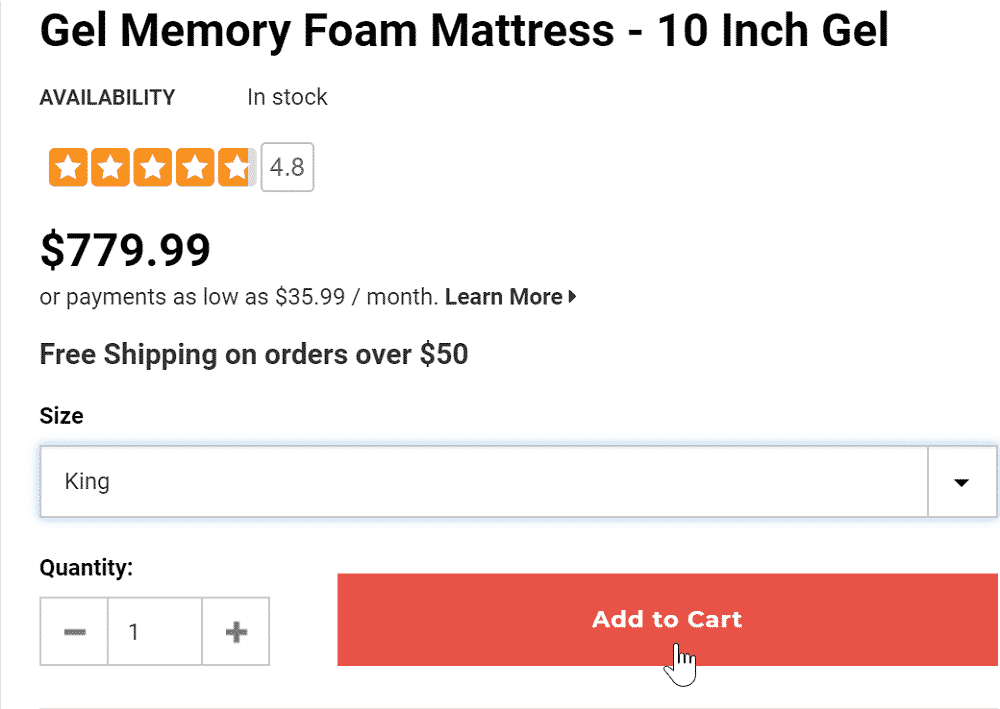"At the top of the image, bold black text reads 'Gel Memory Foam Mattress - 10-inch Gel.' Below this, the word 'Availability' is positioned to the left, and on the right, it states 'In Stock.' Underneath, there are five squares indicating customer ratings. Four squares are completely filled with orange backgrounds and white stars, while the fifth square is mostly orange with a thin vertical strip of gray, showcasing a 4.8-star rating. Next to these squares is the rating '4.8.'

Directly beneath this rating, there's a price tag displaying '$779.99' with a dollar sign, followed by a note that reads 'or payments as low as $35.99/month' with an option to 'Learn more.' Further down, in bold black text, it announces 'Free Shipping on orders over $50.'

Continuing downward, the word 'Size' appears with a selection box underneath containing the word 'King,' accompanied by a downward-pointing arrow indicating a dropdown menu. The section for selecting quantity follows, featuring a negative sign, the number '1' in the center, and a positive sign.

To the right of this quantity selector, there is a prominent red rectangle button labeled 'Add to Cart.' Below this button, an image of a finger pointing upwards directs attention to the 'Add to Cart' area, emphasizing the call to action."